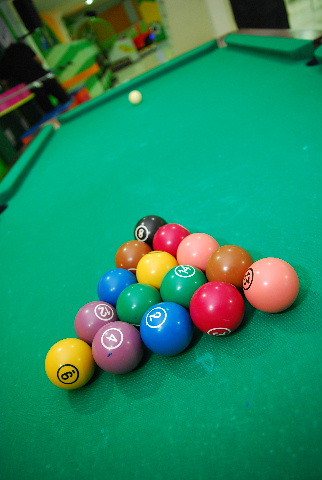This indoor color photograph captures a green felted pool table, slightly angled at 45 degrees to the camera, exuding readiness for play. Central to the image is a neatly arranged triangle of 15 pool balls, comprising two yellow balls, two green balls, two purple balls, two peach-colored balls, two red balls, two brown balls, and a single black eight ball, all drawing clear attention. At the far end, the white cue ball stands poised, awaiting the first strike. The table's wooden trim on the edges suggests a well-crafted design, indicative of use, as evidenced by the faint marks on some of the balls. The foreground is sharply in focus, while the background remains blurry, hinting at possibly being a home game room or recreational center cluttered with indistinct items. This well-composed photograph, devoid of any text, effectively captures the anticipation of an imminent game of pool.